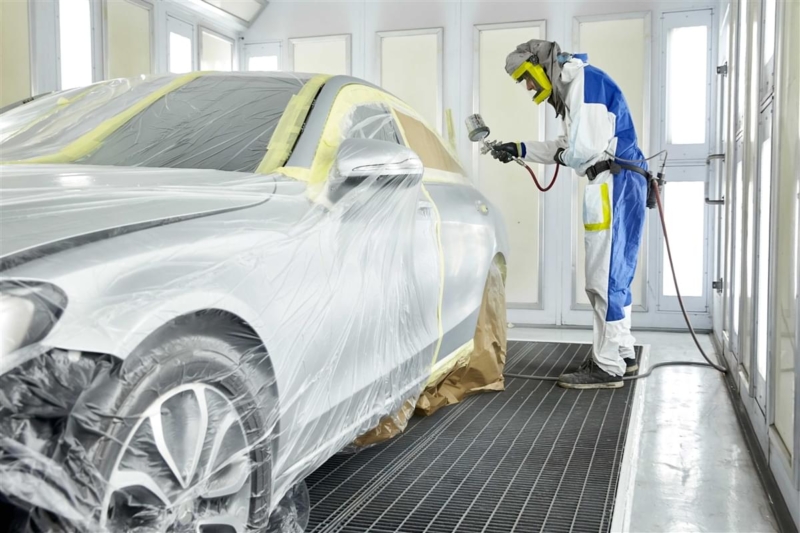Inside a car paint shop, a nearly full-frame car is being prepared for a new coat of paint. The car, oriented with its front to the left, is extensively masked with translucent plastic sheeting, secured along seams with yellow tape and brown paper covering some windows. The vehicle rests on a dark gray grated platform, allowing for drainage. A worker, donned in a blue and white protective suit, complete with a full head mask featuring a clear visor, is actively spray-painting the car using a paint gun extended in one hand. The room itself is enclosed, featuring wide, vertical frosted glass windows that line the walls, creating a controlled environment for the painting process. The car currently exhibits a light silver chrome finish under the protective coverings.